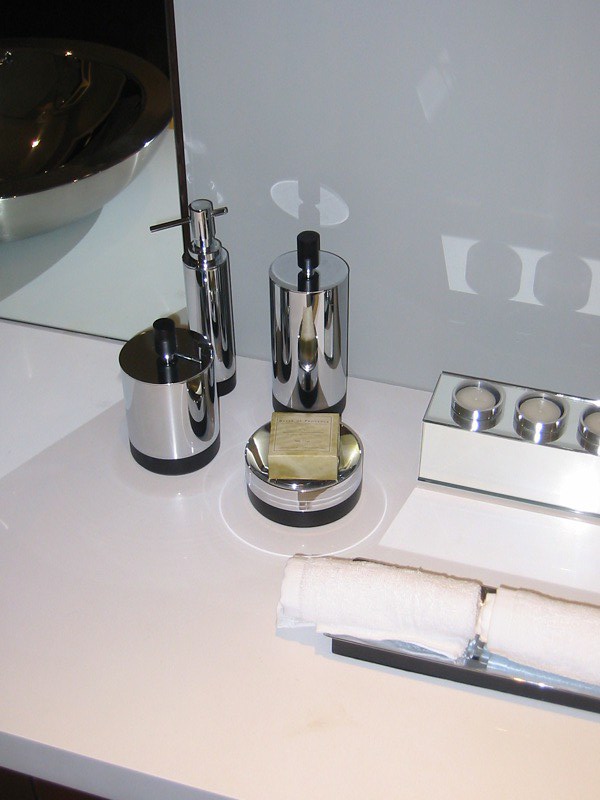The photograph captures an immaculate, white marble countertop with a polished finish. Sitting prominently on the countertop are two neatly rolled white towels perched on an elegant silver stand. In the background, a white rectangular box, featuring a silver top with round cutouts, houses several white tea candles that cast a soft, serene glow. On the left side, a silver circular container with a black bottom holds a square, yellowish-brown object adorned with faint diagonal lines. Adjacent to this is a highly reflective silver cylinder with a black base and a black knob on top. Another slender silver cylinder, just as tall but with a narrower width, stands next to it, showcasing a silver cap with a thin stick protruding through it. At the forefront, a shorter silver container also sports a black bottom and knob. To the far left, a mirror reflects the serene tableau, including a glimpse of a silver bowl, enhancing the overall sense of depth and sophistication in the image.